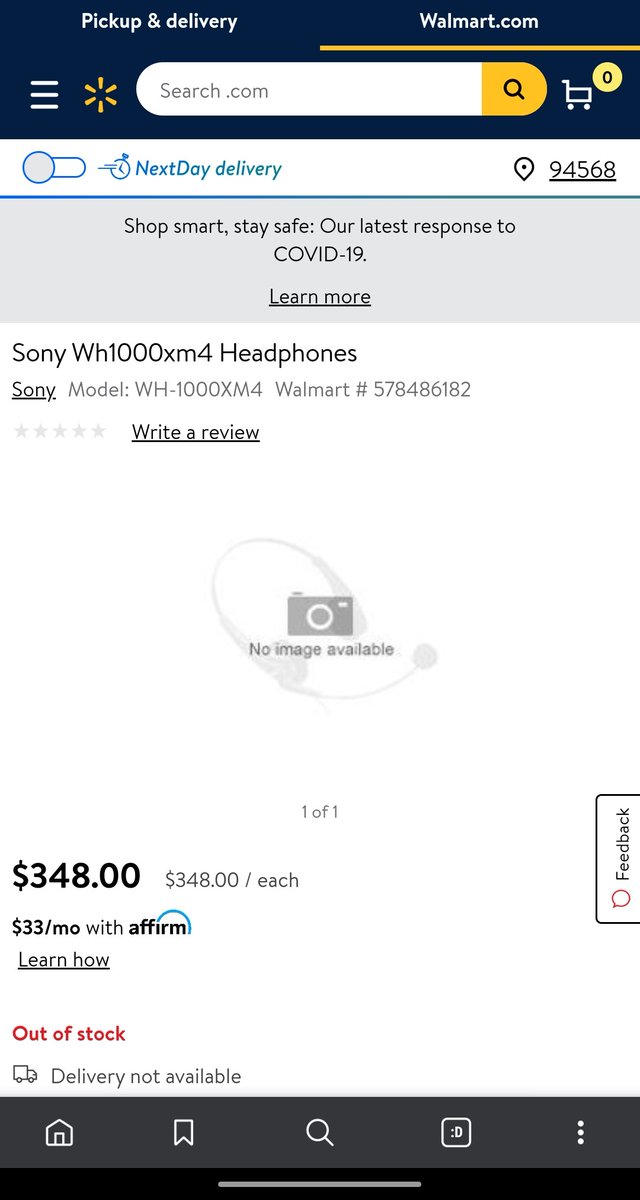The screenshot from the Walmart app features a header predominantly in blue, with "Pick up & delivery" written in white on the left-hand side and "walmart.com" on the right-hand side, underlined by an orange line. To the left, three white lines—indicative of a menu—are visible next to the Walmart logo, which resembles sun rays. 

The interface is divided into two sections: on the left, an all-white field, and on the right, an orange section. Within the white section, "search.com" is inscribed, while a blue magnifying glass icon is present on the orange side. Adjacent to these, there is a white shopping cart icon containing a yellow circle with a blue zero inside of it. 

Below these elements, "Next Day Delivery" is displayed in light blue text, followed by a black "94568" zip code on a thin blue-green line across a gray background. In black text, it reads, "Shop smart, stay safe... Our latest response to COVID-19." Directly beneath this statement, the text "Learn more" is underlined.

The lower section of the screenshot transitions to a white background where the product details are highlighted. It features the text "Sony WH-1000XM4 Headphones" with "Sony" underlined. In light gray, it states "Model: WH-1000XM4, Walmart number: # 578486182." A row of five gray stars is displayed above the prompt "Write a review" in black text. Lastly, the price "$348" is prominently shown.